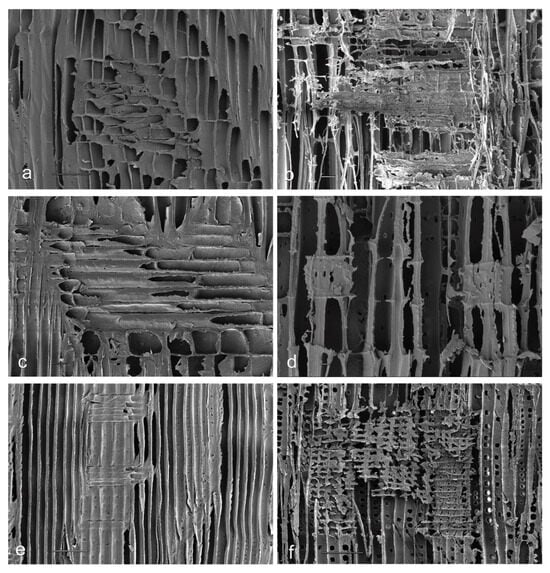The image is a rectangular collage comprised of six separate grayscale photographs showcasing zoomed-in textures, each framed with a thin white border and labeled with a lowercase letter in the bottom left corner of each photo: A, B, C, D, E, and F. The collage is organized into three rows and two columns. 

- Image A, located in the top-left corner, displays tube-like cut-off structures in gray, resembling either foam insulation or rivets in soundproofing material, with an organic appearance similar to cave formations.
- Image B, in the top row next to A, features netting and fabric-like strands that might evoke thoughts of honeycombs due to their intricate, woven texture.
- Image C, positioned in the middle row's first column, appears to show the face of cardboard, characterized by its linear, straw-like slats, reminiscent of cellular or organic structures.
- Image D, next to C, contains sparse vertical stripes interspersed with black gaps, which could suggest a worn or less dense material, possibly an organic fabric.
- Image E, in the bottom-left corner of the collage, has small vertical stripes that might invoke the image of an aged air filter, adding to the organic texture theme.
- Image F, to the right of E, shows something akin to corrugated cardboard with thin circular holes, reinforcing the collage’s overall examination of textured, possibly organic materials.

This intricate arrangement of textures presents a detailed study of various organic and possibly manufactured materials, unified in a black-and-white, microscopic photographic style.